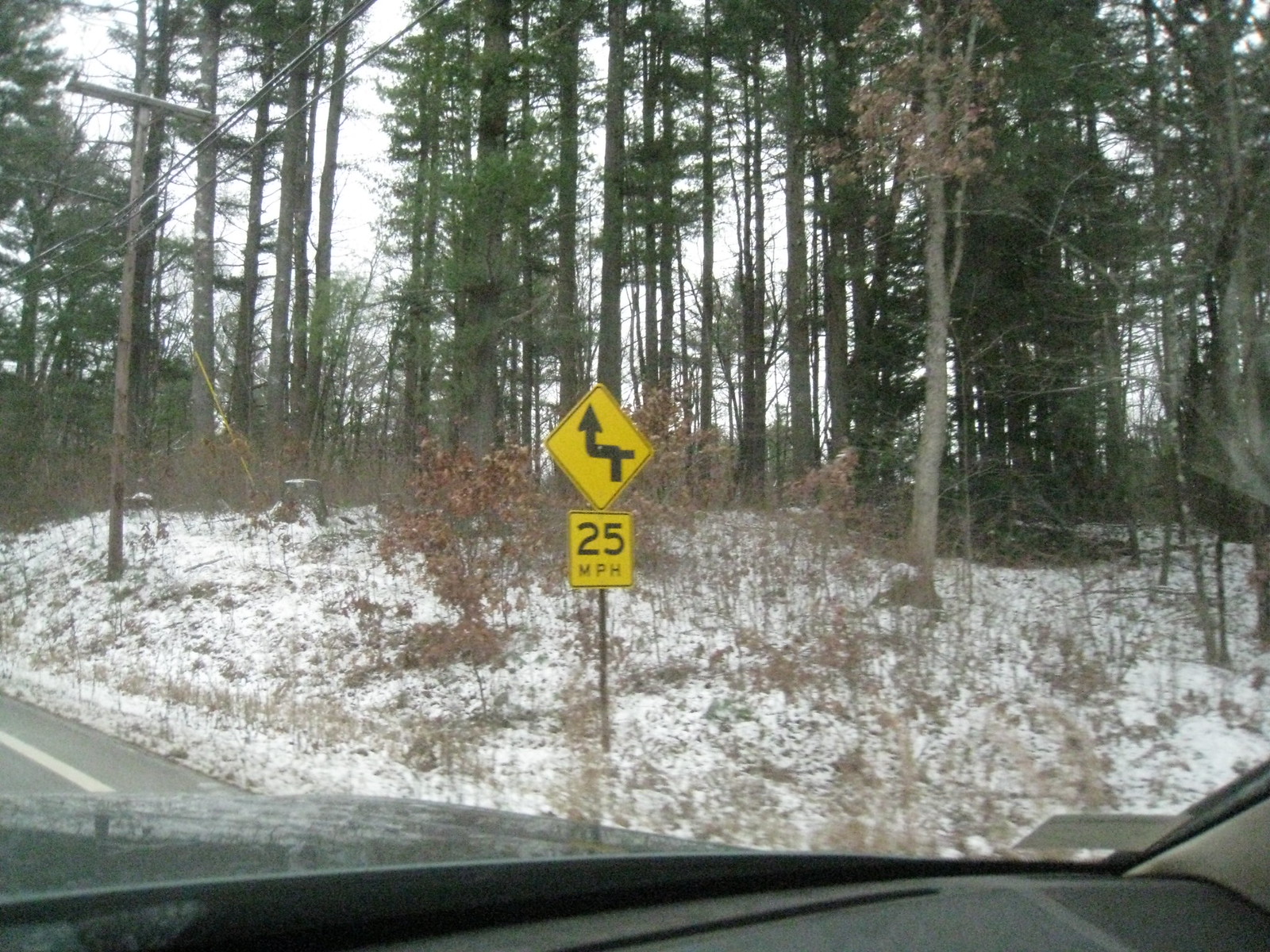The photograph, captured in color from the driver's seat of a car, showcases a winter landscape dominated by snow-covered ground and tall, spindly trees, some possibly pine, extending skyward in the background. In the foreground, brown, dead weeds and branches peek through the snow on a slight hill. The scene features a yellow diamond-shaped road sign centered prominently, displaying a black arrow that curves left and right, indicating a winding road ahead. Directly below it, a yellow square sign reads "25 miles per hour." A telephone pole stands to the left, with electrical wires coming in from the upper left corner. The vehicle's dashboard, hood, and a shadow or reflection of snow on the car's dark roof are visible at the bottom edge of the image. The sky is also partially visible through the treetops.